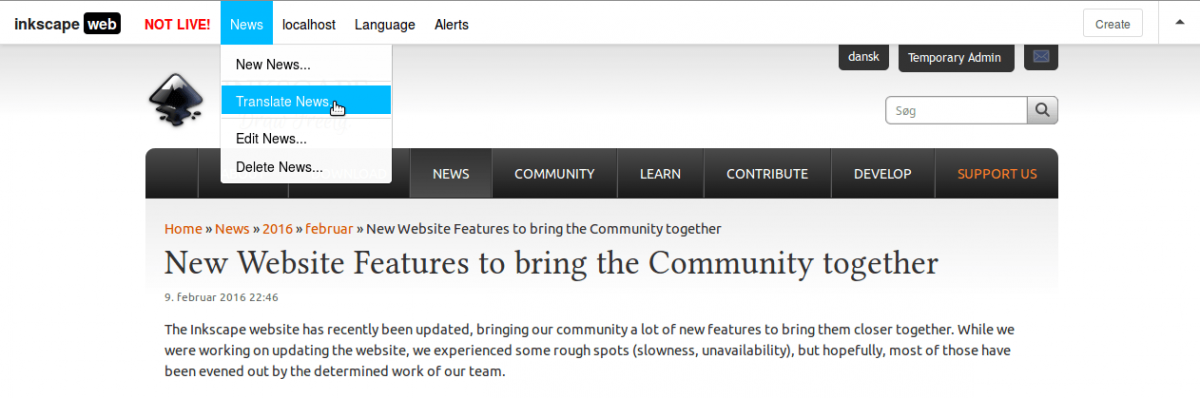This image from the Inkscape website features a predominantly grayish-white background with subtle shades of gray. At the top of the image, the word "Inkscape" is displayed in black. Below it, there are several labels: "Web" with a black background, "NotLive" in all capital red letters followed by an exclamation point, and "News" highlighted in blue. Other categories mentioned include "Local Hosts," "Language," and "Alerts," each accompanied by a dropdown menu. The dropdown menu options under "News" include "New News" and "Translate News," with the latter highlighted in blue and marked with a small, white pointing hand icon. Additional categories such as "Edit News" and "Delete News" are also present.

On the lower right-hand side, "Dansk" and "Temporary Administration" are written in black boxes. In the upper right-hand corner, a white box labeled "Create" with a small arrow icon is visible. A black bar stretches across the width of the screen, featuring menu options in white letters: "News," "Community," "Learn," "Contribute," "Develop," and at the end, "Support Us" in red letters.

Highlighted in red are the words "Home News 2016 February," while the text "New Website Features to Bring the Community Together" is in black. The heading "NEW WEBSITE FEATURES TO BRING THE COMMUNITY TOGETHER" is prominently displayed in all capital letters. Additionally, a timestamp reads "February 9, 2016 at 2246." The accompanying paragraph further explains that the "Lynxscape website has recently been updated, bringing our community a lot of new features to bring them closer together." It also mentions that during the site update, there were challenges (such as slowness and unavailability), but these issues have mostly been resolved through the dedicated efforts of their team. All this explanatory text is written in black.